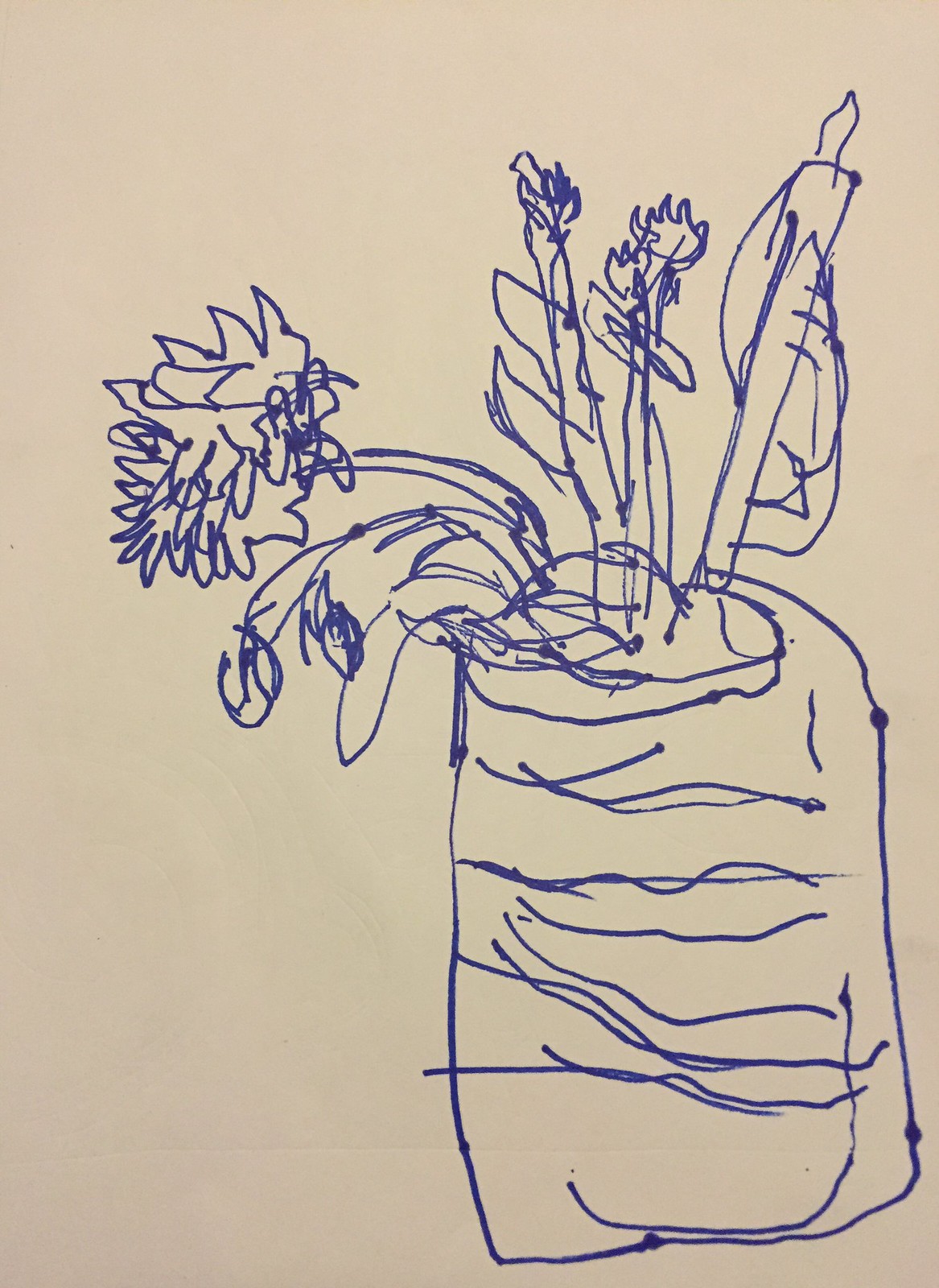This image captures a whimsical pen doodle on a white sheet of paper, depicting a vase filled with flowers. The vase itself is a quirky mix of styles, featuring a semi-straight line on the left side that transitions into a rounded curve at the top of the right side. The surface of the vase is adorned with erratic, squiggly lines that extend from top to bottom, some of which spill outside the boundaries of the vase. Adding to its abstract charm, two dots punctuate the outline on the right—one near the top and the other at the bottom. The base of the vase is noticeably uneven, contributing to its overall child-like, unpolished appearance. 

Inside the vase, the flowers tell their own story of carefree imperfection. Several flowers appear wilted, drooping over towards the left, while two brave stems stand upright on the right. The stems themselves are rendered in jagged, chaotic pen lines, enhancing the rustic, scribbled look of the entire piece. This doodle encapsulates a sense of innocent spontaneity and creative freedom.